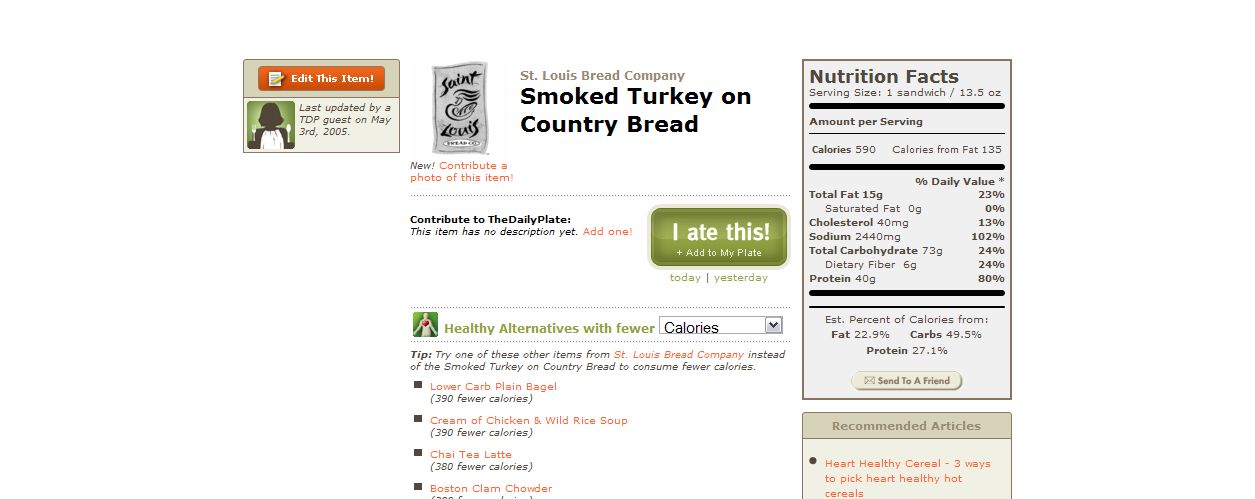The image appears to be a screenshot of an older post from a website called "The Daily Plate," which showcases a food product titled "Smoked Turkey on Country Bread" from the St. Louis Bread Company. The background is white, and in the upper left corner, there is a gray box with a red strip that says "edit this." Below the product title, there is text indicating that it was last updated by a TDP guest on May 3, 2005. There is an "I ate this" button in green, suggesting user interaction. To the right, detailed nutritional facts are presented, including calorie information. Below the main product description, the page offers healthy alternatives with fewer calories, and there are various buttons to modify the page or send the information to a friend. The layout includes drop-down menus for selecting different categories, making it a user-friendly tool for finding and replacing food products for various dietary needs.